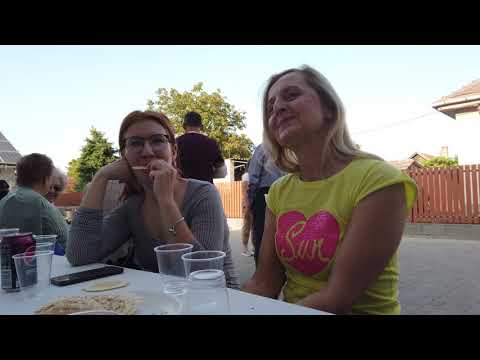The image captures a vibrant outdoor gathering, centered around a white table adorned with a white tablecloth, clear plastic cups, a Pepsi can, a Diet Pepsi, a smartphone, and a plate of food. At the forefront, two women are seated closely, engaging with the scene around them. 

The woman on the right, slightly older, has straight blonde hair cascading just past her shoulders. She is seen wearing a short-sleeved yellow cotton shirt featuring a pink heart in the center with yellow text that reads "sun." Her cheerful demeanor is evident as she smiles softly without showing her teeth. Next to her, on the left, a woman with short red hair and glasses is captured mid-bite, munching on a french fry with her left hand. She sports a long-sleeved, gray ribbed shirt with a scoop neck and accessorizes with a silver bracelet on her left wrist. Her right elbow rests on the table.

The setting extends beyond the main subjects, revealing a lively backdrop. Behind the women, an older couple sits conversing, and several men stand and mingle in a spacious courtyard bordered by a wooden fence. The ground appears to be concrete or gravel, and there's a tree under a clear blue sky, providing a charming outdoor ambiance. The overall scene is framed neatly with a black header and footer, emphasizing the candid, joyful nature of the gathering.